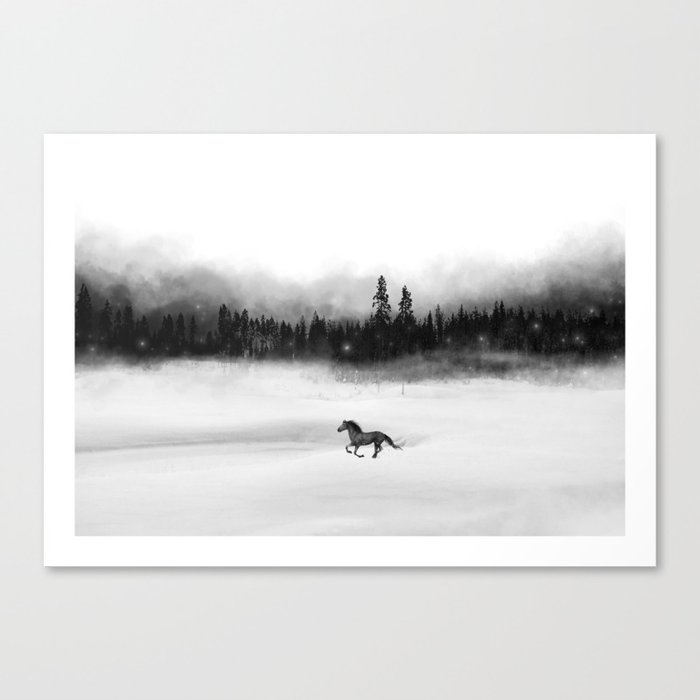This monochromatic image, framed with a white border and mounted on a plain white wall, depicts a lone horse, possibly a wild Mustang, galloping across a snow-covered landscape. The dark horse, which may be brown in color but appears black in this black and white photograph or oil painting, is captured mid-run, facing to the left. The vivid, almost Ansel Adams-like contrast gives the image a lifelike and ethereal quality, enhanced by the dense mist and fog that shroud the landscape. In the background, a row of dark, backlit evergreen trees juts out of the thick mist, with hazy outlines of mountains obscured by clouds. The scene is further accentuated by glowing lights nestled within the trees, adding to the dreamlike atmosphere. The sky, transitioning from foggy to almost pure white as it ascends, completes this serene and evocative winter tableau. The image is landscape-oriented, longer than it is tall, and may appear on canvas or as a high-quality print.